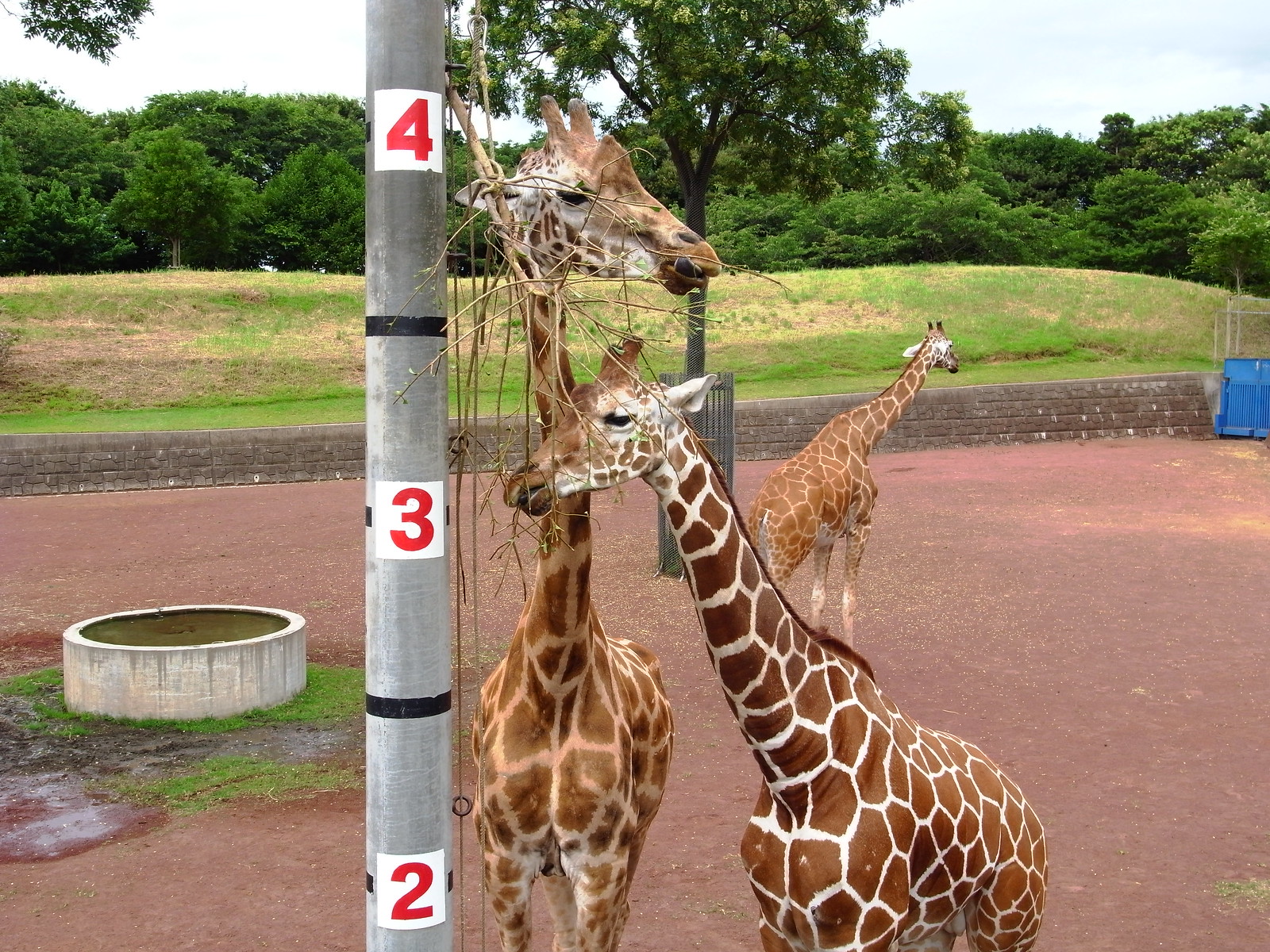The image depicts a high-quality photograph of an outdoor enclosure, likely in a zoo or protected habitat, containing three giraffes. The setting features a stone or brick retaining wall with green grass and a line of trees ascending a small hill in the background. In the enclosure's foreground, there is red dirt or clay, along with a tall metal pole marked with measurements—specifically meters, as indicated by red-font numbers two, three, and four on a white background with black stripes in between.

The two giraffes positioned at the front of the image are standing beside this pole; one giraffe, approximately four meters tall, is on the left and is chewing on tree branches, while the other giraffe, around three meters tall, is to its right, also engaged in eating the branches. To the left of these giraffes is a circular concrete structure, presumably a watering trough. On the right side of the enclosure, a blue gate or bin is visible.

In the mid-ground of the photo, there is a tree encased by a small fence, and further back, the third giraffe stands with its back to the camera, facing toward the blue gate. The sky above is white, providing a clear backdrop to the scene. The image captures the serene, naturalistic environment designed for the giraffes, highlighting both the animals and their habitat in fine detail.